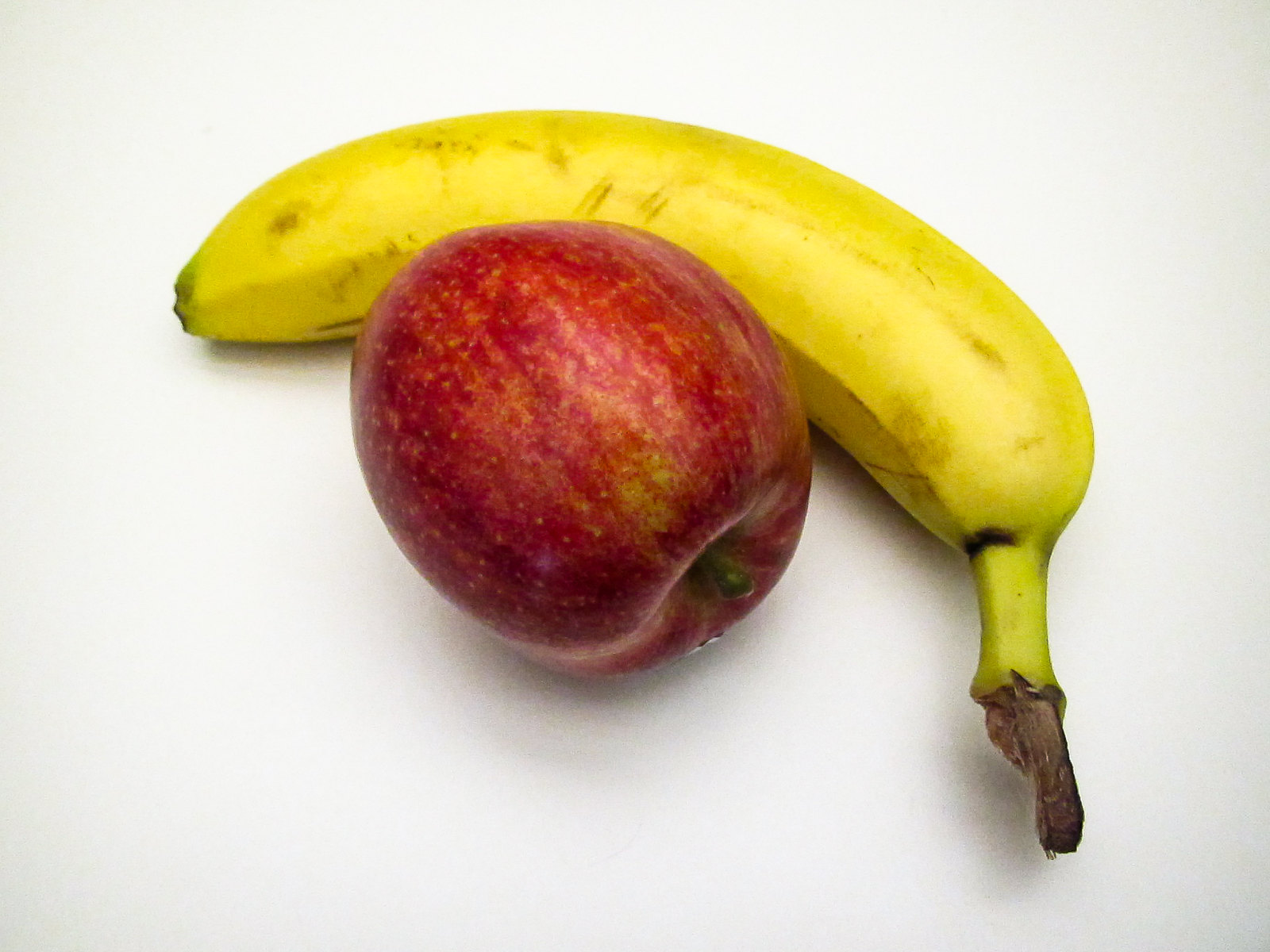This horizontal rectangular photograph features a clean white background with two prominently displayed pieces of fruit: a banana and a red apple. The banana's stem is positioned toward the bottom right edge of the image, approximately a quarter of the way up from the bottom. The stem is brown, transitioning into a yellow segment before the banana itself begins, which starts midway down the right side and curves elegantly towards the left side, ending slightly more than a third away from the left edge. The vibrant yellow banana showcases a few brown markings, adding a touch of realism.

Nestled within the curved embrace of the banana is a deep red apple. The apple's stem points towards the lower right corner, contrasting with the banana stem, which points directly downward. The apple features a tiny green spot and appears to have a partially visible sticker on the far side. Subtle shadowing beneath both the apple and the banana adds depth to the image, enhancing the fruits' natural contours.